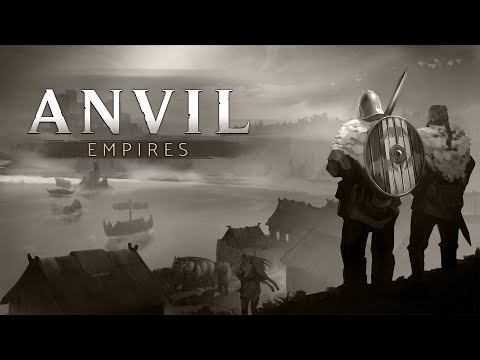This detailed digital painting, a promotional poster for the game "Anvil Empires," showcases a foggy medieval scene dominated by earthy tones of dark brown and gray. The image features two predominant Viking-like soldiers on a hill overlooking a body of water teeming with warships and boats. The soldier on the left has a silver helmet, a circular wooden shield adorned with a white stripe on his back, and wields a sword. Draped in a large fur-lined collar, he stands beside another warrior with a ponytail, sporting similar fur attire and a half cape. This second warrior also has a sheathed sword at his side. Below them, a shanty village with straw-roofed huts can be seen extending toward the fog-covered water, which emits a dense mist that obscures the far-off buildings on the opposite shore. The logo "Anvil Empires" is prominently displayed in the top left-hand corner, completing the atmospheric visual.